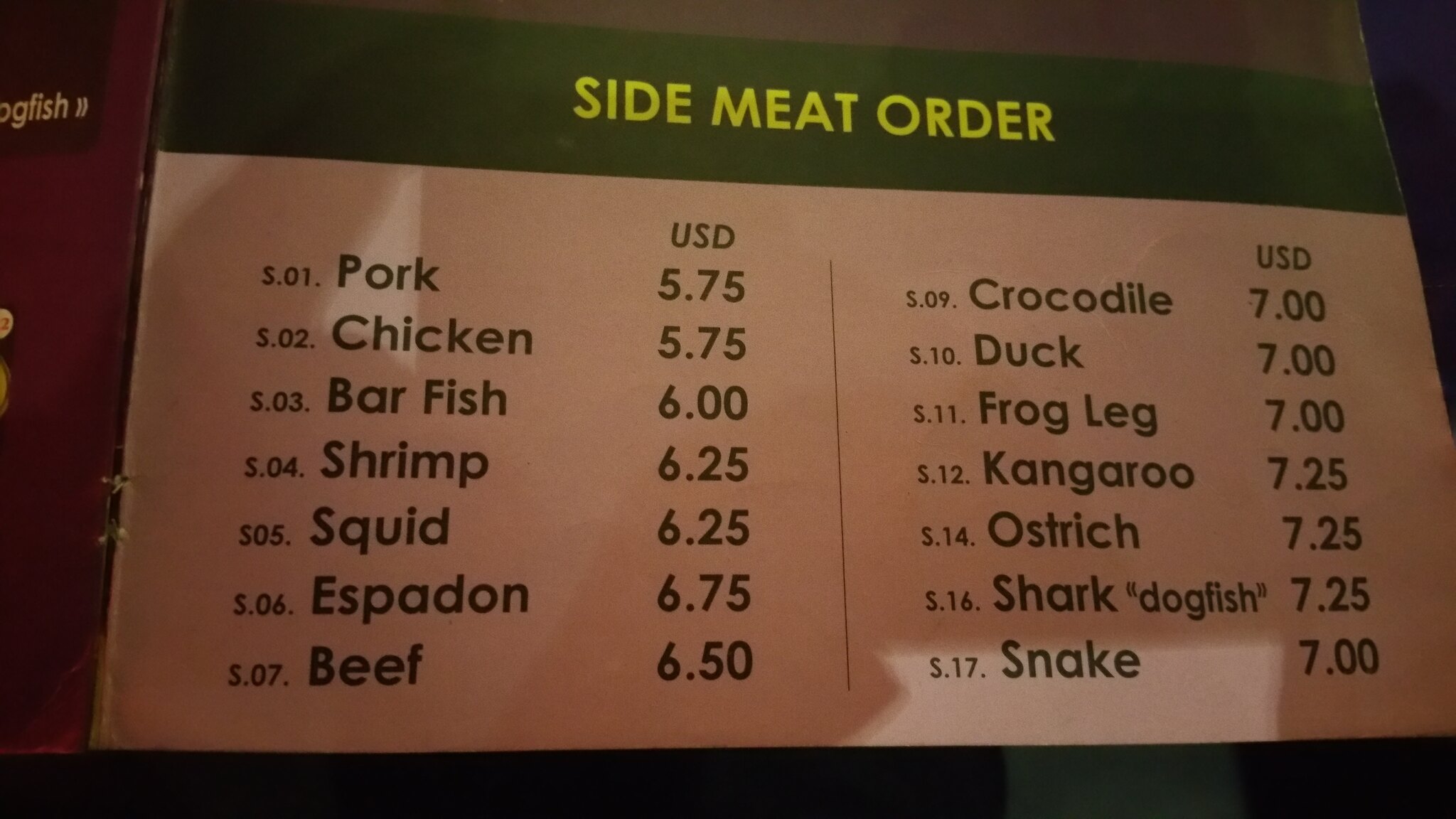The image depicts a portion of a menu, specifically listing options for side meat orders. At the top, the title "Side Meat Order" is prominently displayed in yellow text against a green background. The menu is divided into two columns, each featuring a series of meat options, all priced in US dollars.

On the left side, the options are labeled from S.01 to S.07:

- S.01 Pork - $5.75
- S.02 Chicken - $5.75
- S.03 Barfish - $6.00
- S.04 Shrimp - $6.25
- S.05 Squid - $6.25
- S.06 Espadon - $6.75
- S.07 Beef - $6.50

On the right side, the numbering starts at S.09 and goes up to S.17, with some numbers skipped (notably S.08, S.13, and S.15). The seven options listed here are:

- S.09 Crocodile - $7.00
- S.10 Duck - $7.00
- S.11 Frog Leg - $7.00
- S.12 Kangaroo - $7.25
- S.14 Ostrich - $7.25
- S.16 Shark Dogfish - $7.25
- S.17 Snake - $7.00